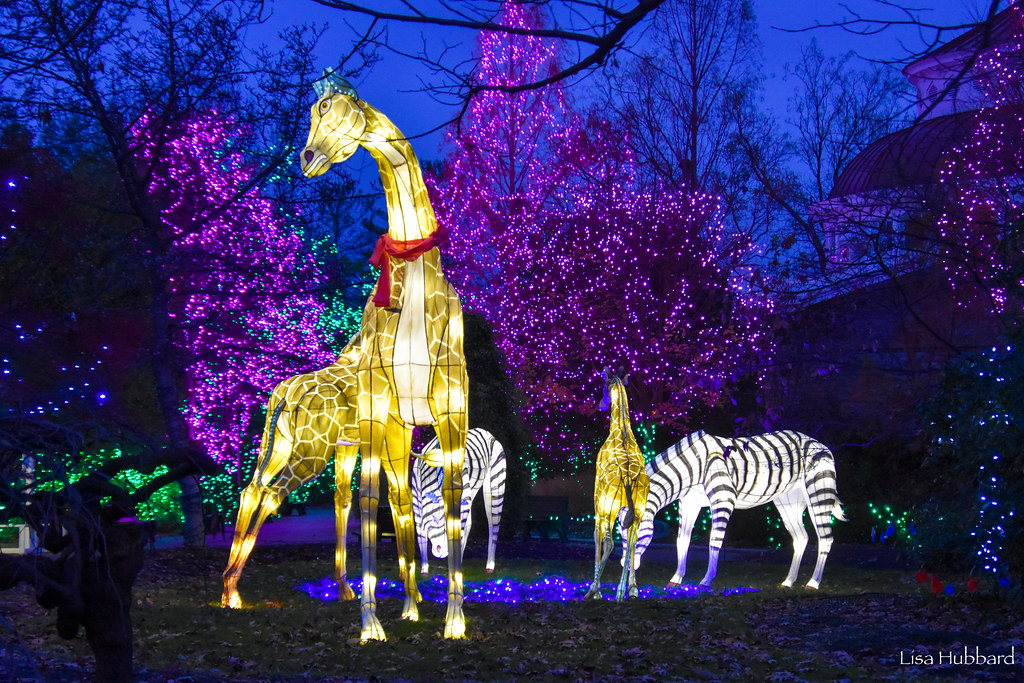The image captures an enchanting outdoor light display at a zoo, likely during Christmastime. The scene is set in the evening, casting a dark, almost purple hue over the sky that hints at the recent dusk and outside lighting. In the far background, leafless trees stand with their bare branches silhouetted against the sky. Closer to the viewer, trees adorned with twinkling purple lights create a magical atmosphere, interspersed with vibrant green lights.

In the foreground, an artistically lit giraffe takes center stage. There appears to be a second giraffe positioned behind the first, causing an intriguing optical illusion of a single giraffe with too many legs, suggesting the presence of another giraffe subtly superimposed. Further back, two zebras are illuminated, adding to the festive zoo-themed display. Additionally, another giraffe is visible in the distance, this one facing away from the viewer, with only its tail discernible. The image is credited to Lisa Hubbard, as indicated in the photograph.